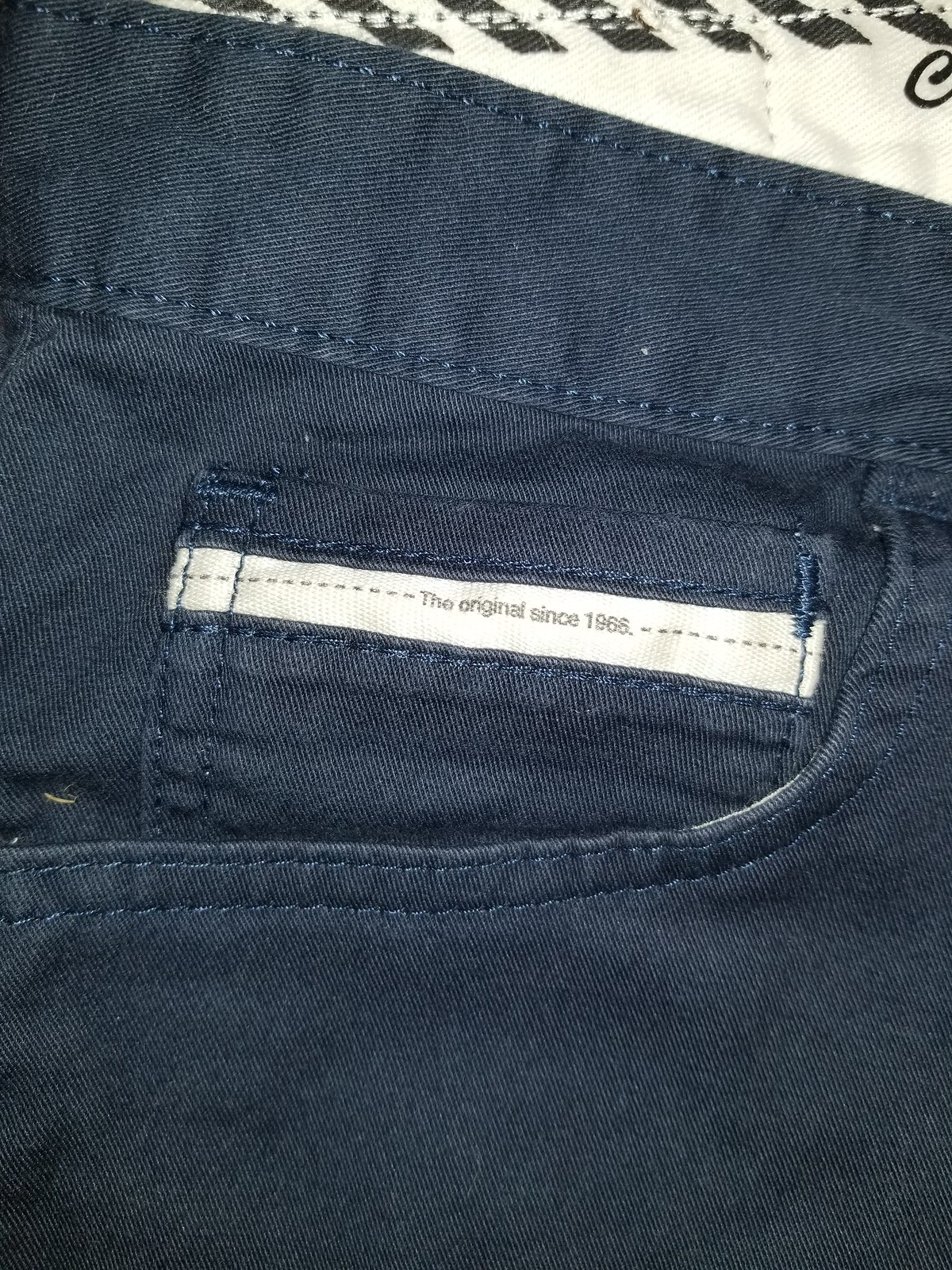This is a close-up color photograph of a dark blue, diagonally-patterned denim fabric, depicting a central pocket on a pair of pants. The pocket includes an internal, square-shaped mini-pocket, which is also dark blue. Centered at the top of the mini-pocket is a white, horizontally placed rectangle label with black text that reads, "The Original Since 1985." The label features dotted lines through the middle in black. Above the pocket, towards the upper right-hand corner of the image, there is a glimpse of a contrasting white fabric, believed to be part of a quilt or the inside lining of the pants, adorned with black emblems or decorative hash marks. Additionally, part of the letter "C" is visible within this white section, hinting at further design or branding.